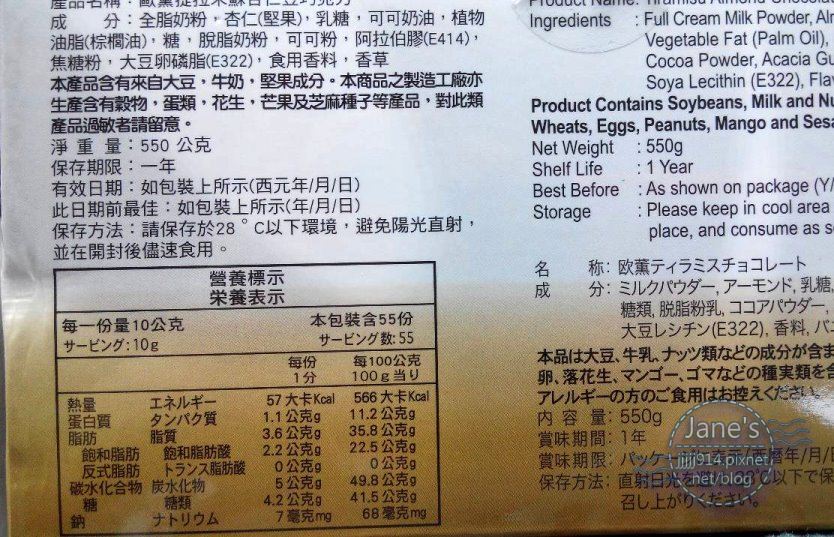This detailed close-up photograph captures the back of a food package prominently featuring a nutritional label primarily in Asian pictograph figures. The entire left side of the label displays these characters, with a few exceptions where some readable numbers and kilocalories are noted. A section of the label is distinctly boxed off. Partial visibility on the right side reveals an ingredients list in the top right corner, including full cream milk powder, vegetable fat, cocoa powder, and soy lecithin. Notably, the product contains allergens such as soybeans, milk, wheat, eggs, peanuts, and mango. The total weight is specified as 550 grams, with a shelf life of one year. A watermark in the lower right corner reads "Jane's 914 PixNet/blog."